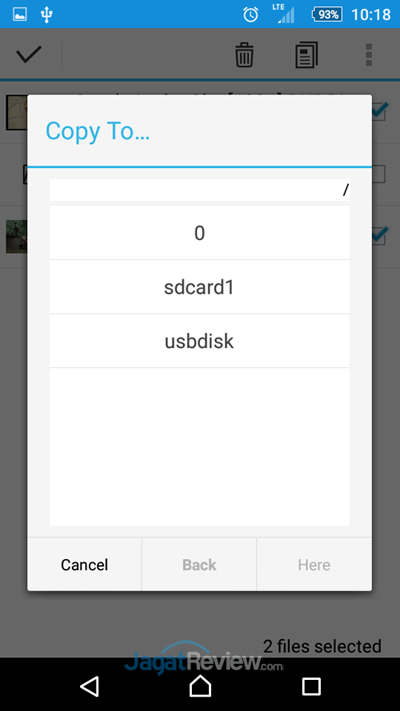The screenshot features a vibrant blue header spanning the upper inch of the screen, setting a striking backdrop. On the far left, there's a small box icon with a miniature USB symbol adjacent to it. Moving rightwards, a clock displays the time as 10:18, though it is unclear if it is AM or PM. Next to the clock, a battery icon indicates a robust charge level of 93%. However, the LTE signal strength is weak with only one bar illuminated. 

Beneath the header is a sizable white box that reads "copy 2" underlined with a blue line. Below this, it lists "zero SD card," "one USD disk," and mentions that two files are selected. At the bottom of the screen, a black bar runs horizontally, containing a home symbol, a square icon, and an arrow pointing to the left. The overall layout appears organized yet functional, highlighted by the contrasting colors and icons indicating various statuses and functions.